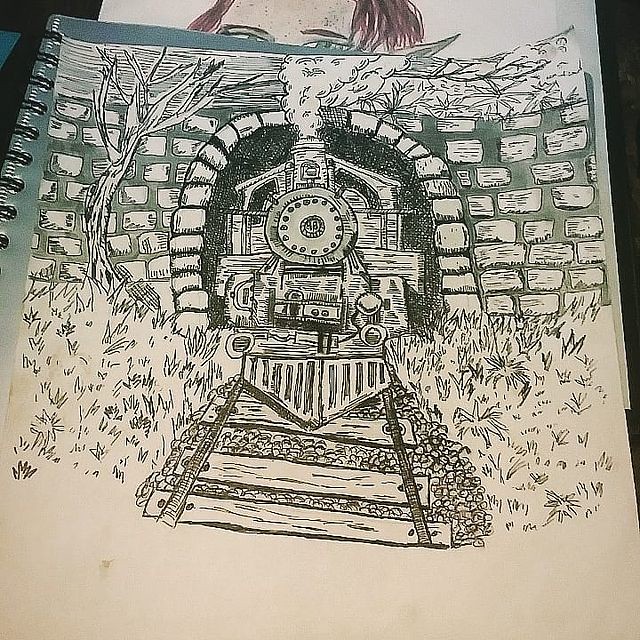The image showcases a detailed sketch set against a dark-colored tabletop. A black-bound sketchbook with a green cover lies at the center. On top of this sketchbook is a piece of torn sketching paper featuring an elaborate drawing of a steam train engine emerging from a tunnel. The tunnel entrance, crafted from stone bricks, stands against a dark, circular backdrop that accentuates the train's emergence. The scene is enriched with small but intricate details: a leafless tree stands starkly beside the tunnel's broken brick wall, and grass surrounds the train tracks. Wisps of smoke trail from the train’s funnel, painstakingly shaded to enhance the realism. Beneath the sketchbook, the edge of another sketch peeks out, revealing part of a person's face with brown hair and green eyes. This dual-layer composition invites viewers to appreciate the artistry and meticulous effort put into both sketches.